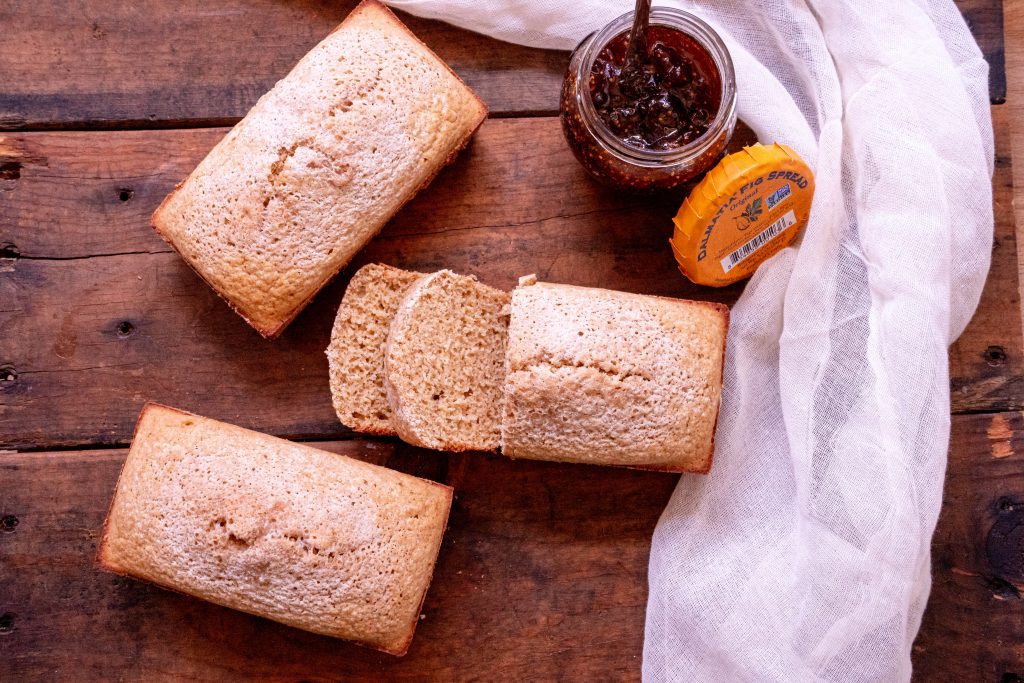The photograph depicts a rustic scene of a dark brown wooden picnic table adorned with three freshly baked loaves of bread. On the left side of the table, two whole loaves frame a third loaf that has two slices cut from it. The bread resembles a dense, risen variety, possibly banana bread or a similar cake-like bread. To the right of the loaves, there is an open jar of dark jam or spread, likely a fruity confection like cherry or blueberry jam, with an orange lid. The brand name on the jar isn't visible. Draped across the right side of the table is a thin, white, diaphanous cloth that winds around the jar and extends towards the bottom of the image, adding a soft, airy contrast to the rustic wooden texture and the hearty loaves of bread.